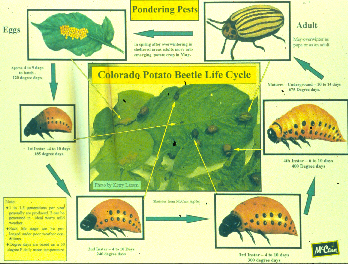This image is a detailed textbook illustration depicting the life cycle of the Colorado potato beetle. At the center, amidst a green and yellow background, the title "Colorado Potato Beetle Life Cycles" is prominently displayed. Surrounding the central image are six smaller drawings, each representing a different stage in the beetle's life. The cycle is arranged counterclockwise, beginning at the upper left with the yellow eggs attached to a leaf, progressing to the larval stages on the lower left, continuing to a more mature larva at the bottom, and culminating at the upper right with the illustration of an adult beetle. The adult beetle is characterized by its yellow body with horizontal black stripes, six legs, two antennae, and a black head and legs. Green arrows connect each stage, visually guiding the viewer through the beetle's developmental process. Additionally, the lower left corner of the image contains a yellow square with written narrative explanations to enhance understanding. The overall color scheme features green, yellow, and black, providing a clear and visually engaging representation of the beetle's life cycle.